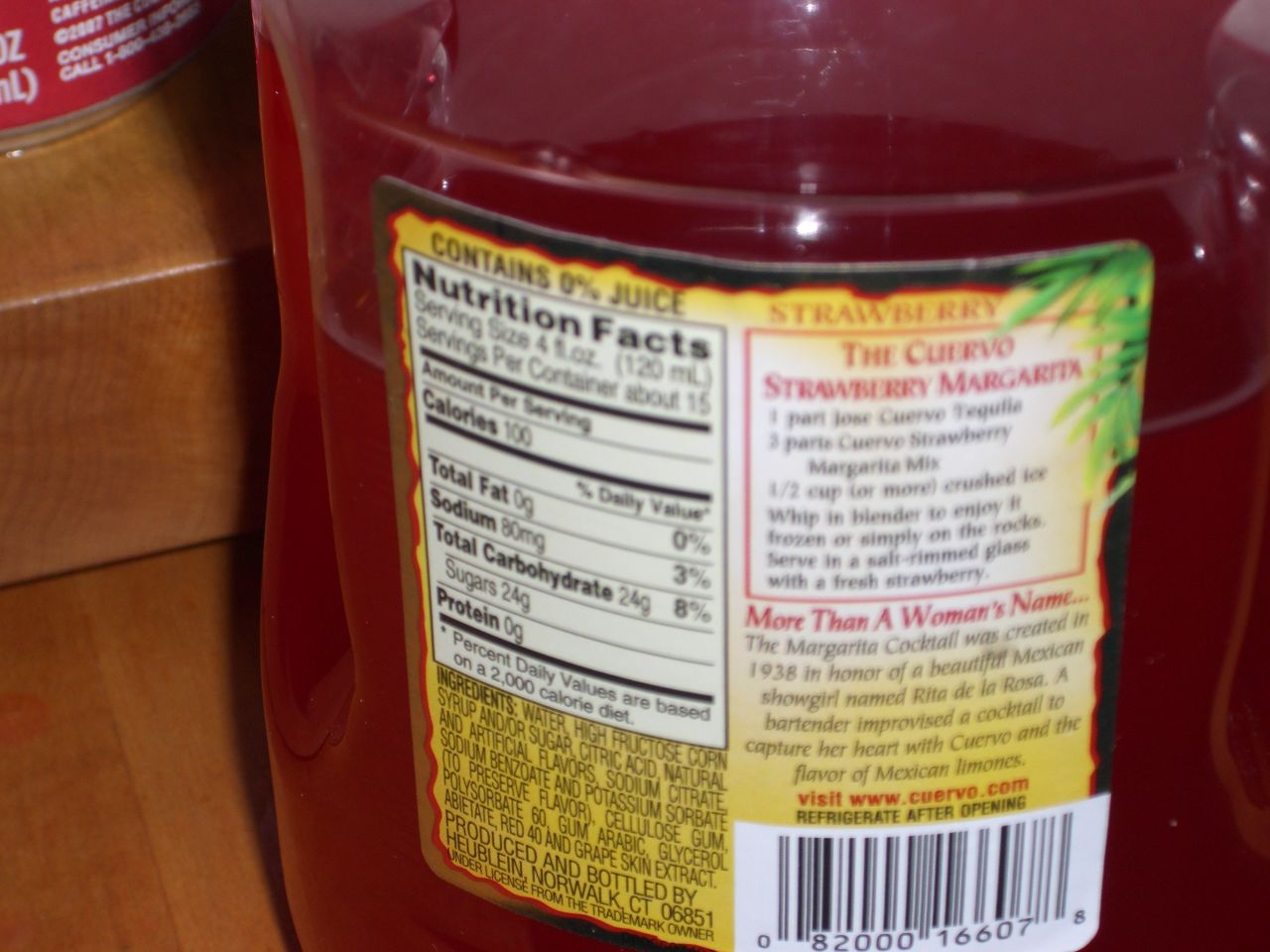The image depicts a large plastic container filled with a red liquid, placed on a dark brown wooden table. The container is shown from the back and features a detailed label. The label is predominantly yellow with black, brown, and green borders, and includes a barcode at the bottom right. Above the barcode, on the left side, are ingredients and a nutritional facts table which indicates the drink contains 0% juice and has 100 calories, 8% carbohydrates, and 24 grams of sugar. The right side of the label features the words "Strawberry" and "Margarita" with a Cuervo strawberry margarita recipe. The label also recounts the origin of the margarita cocktail, stating it was created in 1938 by a bartender to capture the heart of a beautiful Mexican showgirl named Rita de la Rosa. The bottle includes instructions to "Refrigerate after opening" and has a cut-out design for easy gripping. The photograph, taken with a flash, shows a reflective light on the plastic, and there is what appears to be a red can with white writing near the top of the frame.